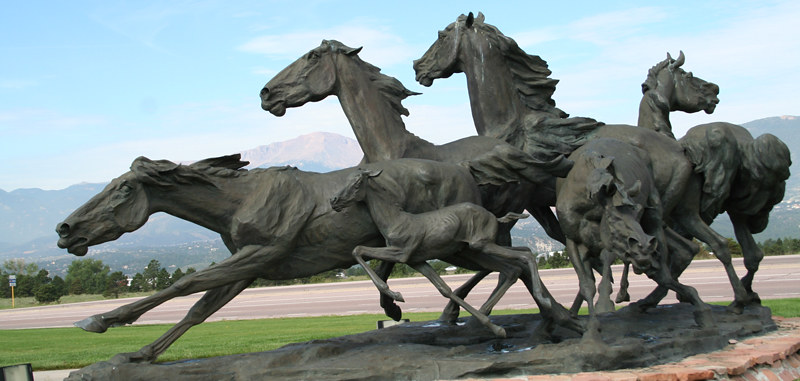The image depicts a dynamic statue of six horses, consisting of four adult horses and two foals, all captured in full motion. The horses, seemingly made of dark gray metal, exhibit detailed musculature and flowing tails, with some racing towards the left while others appear poised to dash in different directions. The statue rests atop a substantial brick pedestal set in an open field. In the background, a maintained dirt horse racetrack stretches from left to right. Beyond the track lies a highway bordered by patches of grass and short trees, leading to a tree-lined valley and a range of majestic mountains. The sky above is light blue, partly cloudy, and adds a serene backdrop to the scene. Also faintly visible are specks of a distant city, enhancing the picturesque quality of the landscape.